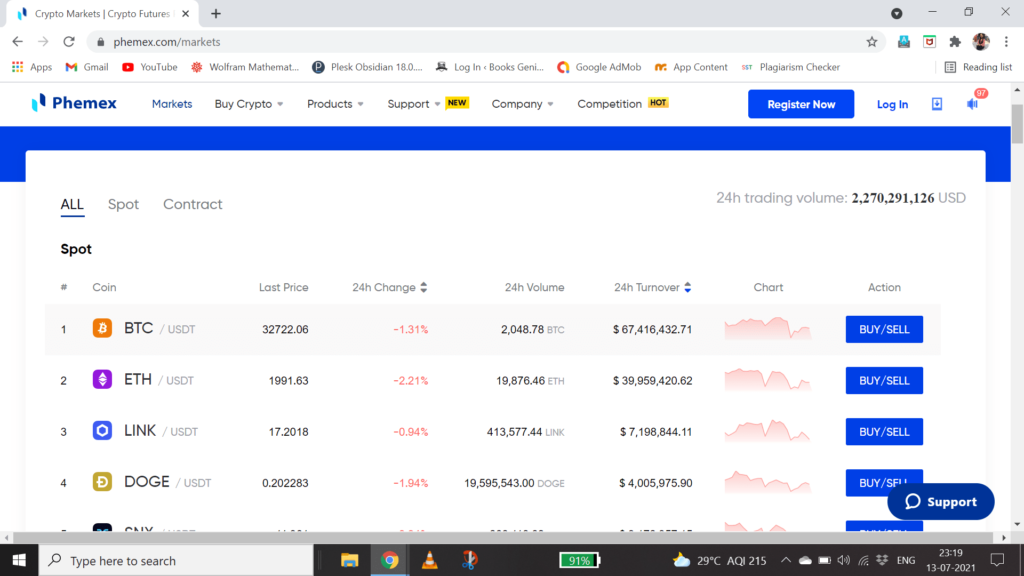In this image, we see a detailed screenshot of a webpage displaying a list of cryptocurrencies and their respective prices. The interface at the top features a search bar and various navigation buttons for apps, Gmail, YouTube, and other services. Additionally, the browser window controls, including the close (X), minimize, and tab buttons, are visible at the top right, with the active tab located at the top left.

The main content area showcases the list of cryptocurrencies against a clean, white background. Each cryptocurrency is accompanied by its company logo to the left and its name in black text to the right. The cryptocurrencies are ranked and listed as follows: 
1. Bitcoin
2. Ethereum
3. Link
4. Dogecoin

On the far right of each cryptocurrency row, there is a prominent blue "Buy/Sell" button. Adjacent to this, towards the left, the 24-hour turnover for Bitcoin is highlighted, showing an impressive $67 billion. Additional columns provide detailed stats including a 24-hour volume and a 24-hour change, with Bitcoin specifically noted to have decreased by 1.3% over the last 24 hours.

At the top right corner of the webpage, a 24-hour trading volume indicator displays a substantial figure of $2,270,000,000 USD traded, offering a comprehensive snapshot of the current trading activity.